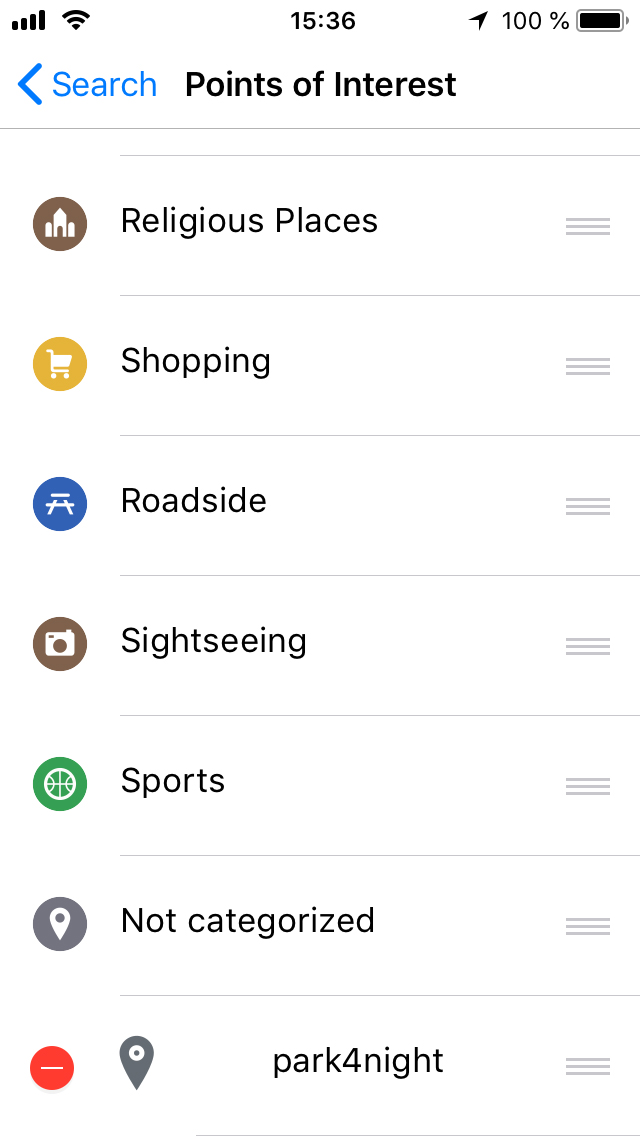This image, displayed on an Apple smartphone, features a clean white background. At the top left corner, the word "Search" appears in blue text. The top portion of the screen prominently displays the title "Points of Interest". Below this header, there are seven categorized points of interest, each accompanied by a distinct circular icon on the left.

1. **Religious Places**: The icon is brown, depicting a white church.
2. **Shopping**: Represented by an orange icon featuring a white shopping trolley.
3. **Roadside**: This category has a blue icon with a white railway line.
4. **Sightseeing**: Indicated by a brown icon with a camera design.
5. **Sports**: The icon for this category is green, showcasing a white basketball.
6. **Not Categorized**: Marked by a grey icon with a white location pin.
7. **Park Night**: The icon is red, featuring a minus sign. To its right, there is a grey location pin icon with a small white circle inside.

Each category is accompanied by three black horizontal bars on the right side, allowing users to sort them.